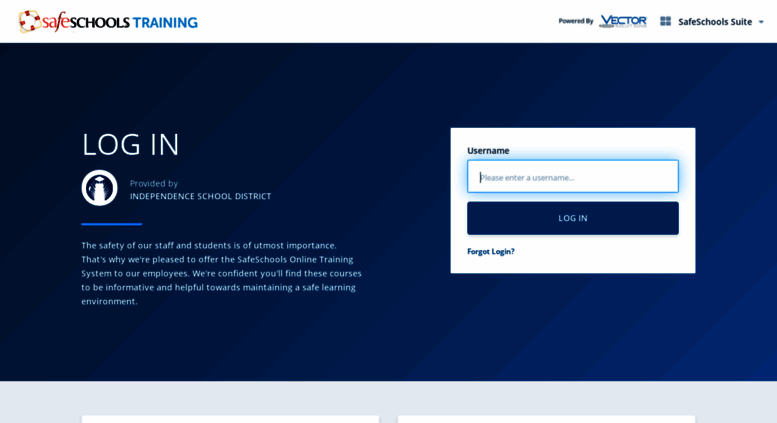The image is a screenshot of the Safe Schools Training website, designed for school faculty and staff to access training resources for maintaining a safe school environment. 

**Top Left Section:**
- **Logo and Text:** The site’s name, "Safe Schools Training," is displayed prominently. The word "Safe" is in red, "Schools" is in black, and "Training" is in blue. Accompanying the text is the website's logo, a small red and white buoy, symbolizing safety and rescue.

**Top Right Section:** 
- **Powered by Vector:** An icon indicating that the website is powered by Vector, a web technology platform. 
- **Safe Schools Suite Dropdown:** A dialog box labeled "Safe Schools Suite" with a downward arrow allows users to navigate to different sections of the website.

**Center Section:**
- A large, dark blue box dominates the center of the screen.
  - **Login Information:** On the left side, in white text, are instructions for logging in. It indicates that access is provided by the Independence School District.
  - **Paragraph about the Site:** Below this, a paragraph explains the importance of the site. It reads, “The safety of our staff and students is of utmost importance. That’s why we’re pleased to offer the Safe Schools Online Training System to our employees. We’re confident you’ll find these courses to be informative and helpful towards maintaining a safe learning environment.”
  
**Right Side of the Center Section:**
- **Login Fields:** A white box where users can enter their username and password to log in. A blue login button is located directly below these fields.
- **Forgot Login Option:** At the bottom of this box, there is a small blue text link labeled "Forgot Login," which users can click if they need to recover their account details.

Overall, the screenshot provides a detailed view of the Safe Schools Training website’s main features and login process, emphasizing its role in promoting safety through online training for school districts.